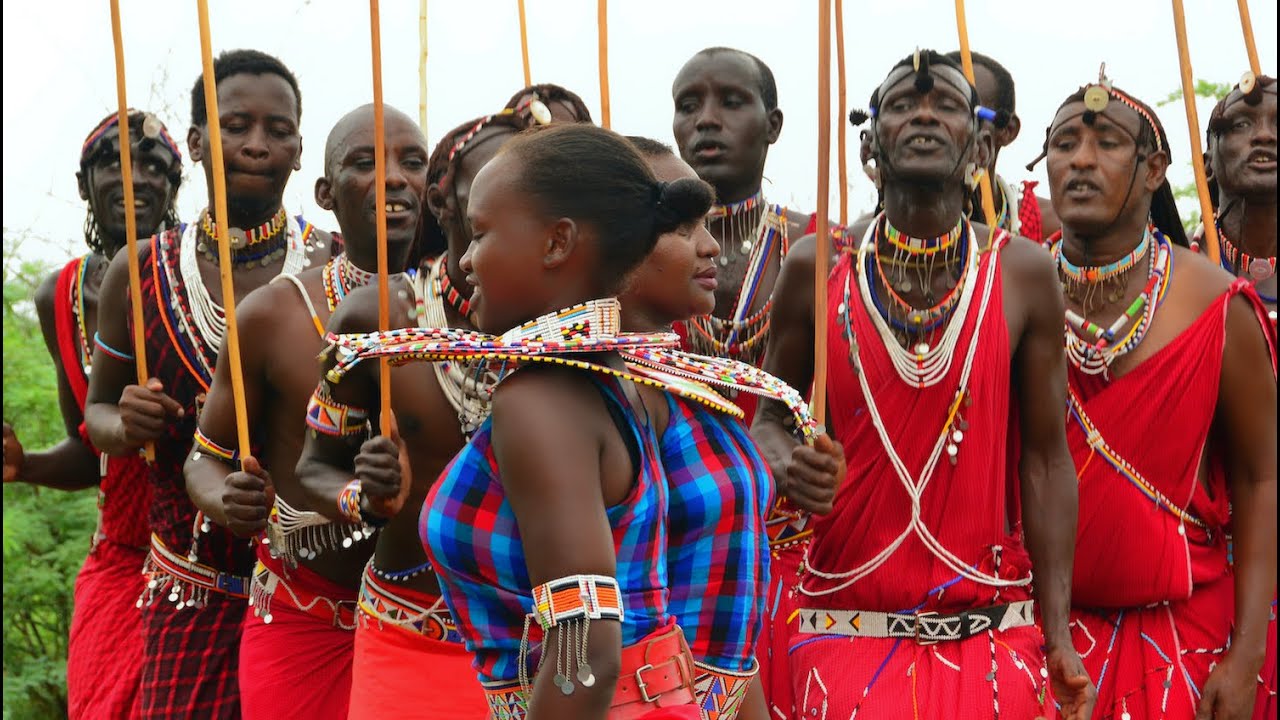The photograph features a group of people who appear to be members of an African tribe, characterized by their similar attire and intricate jewelry. The men, who have rich dark brown skin, are primarily dressed in red outfits resembling tank tops paired with skirts or pants. A few, however, are shirtless or wear bright blue plaid tops. All the men have relatively short hair or are bald and are holding thin, smooth sticks in their right hands, extending above their heads. The men's belts are decorated with light tan colors and ornate beading. In the foreground, two women wearing large, elaborate neck ornaments that extend outward are interlocking arms, with one woman looking to the left and the other to the right. The men in the background are observing the women and uniformly holding their sticks, which could be wooden dolls or spears.